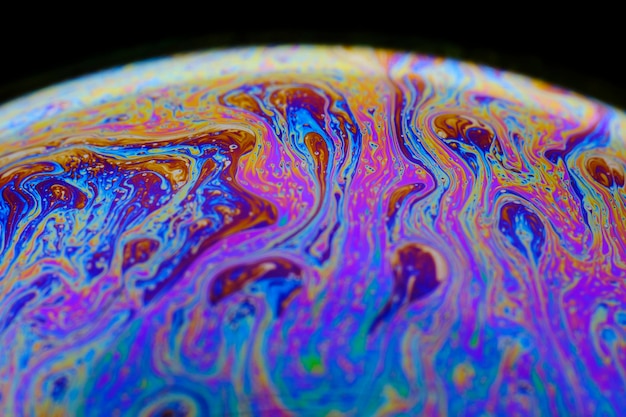This image features a vibrant, abstract depiction of a curved, spherical surface with a dark black background at the top. The surface is covered with intricate, brightly colored patterns that weave throughout, resembling swirling carvings or lines. The colors range from fluorescent green, turquoise, and darker blue to orange, red, yellow, pink, and purple, creating an illuminated, almost neon effect. The colors appear to flow together like mixed paint or swirling oil, becoming darker and larger towards the bottom of the image. The top of the image is notably pitch black, enhancing the reflective and shiny appearance of the colored patterns. The abstract nature of the design, with its high-contrast, psychedelic colors and lack of a clear pattern, evokes images of either the upper atmosphere of Earth with specialized lighting or an artistic interpretation of a cosmic or surreal scene.